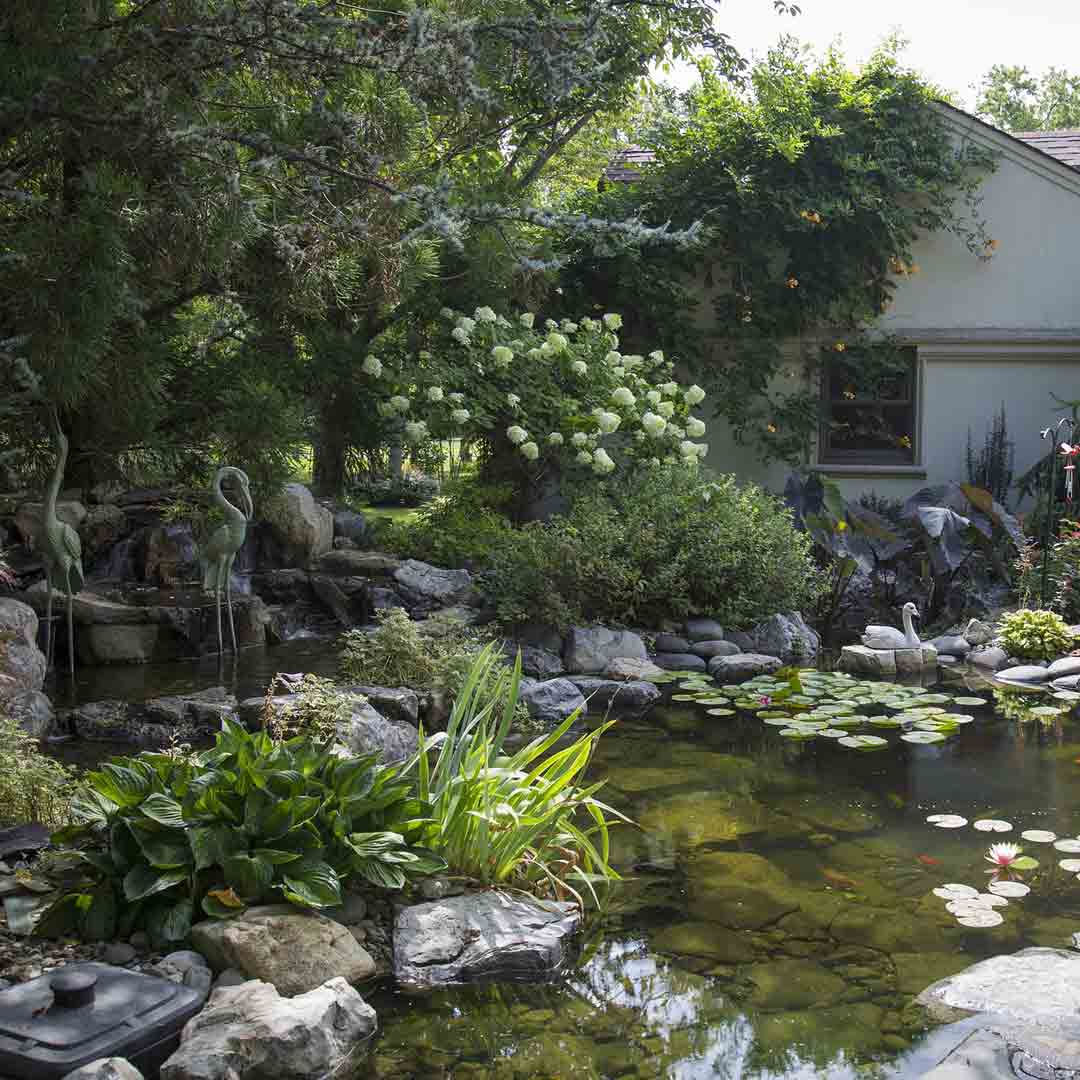The image depicts a picturesque fish pond situated alongside what appears to be an older, possibly gray, garden cottage or ranch-style house covered in blossoming ivy. The pond, approximately 15-20 feet across, has a murky but natural appearance with numerous floating lily pads. Its clear water reveals orange goldfish swimming among the stones at the bottom. Adorning the pond are a series of statues: a white swan poised gracefully on a rock, and two iron statues of cranes or herons, each in distinct poses—one with its beak pointing upwards and the other downwards.

The perimeter of the pond is lined with an abundance of rocks and diverse water plants, including grasses well-suited to the humid environment. On the grounds surrounding the pond, there are sizable trees, one potentially being an orange tree, adding to the lushness of the scene. Near the pond's edge, close to the house, stands a blooming hydrangea plant. Additional foliage, including what appears to be a rose bush, contributes to the vibrant plant life. The cottage's window overlooks this delightful water feature, framed by a stunning backdrop of verdant trees and an assortment of brightly colored, blossoming flowers that lend a sense of tranquility and beauty to the setting.